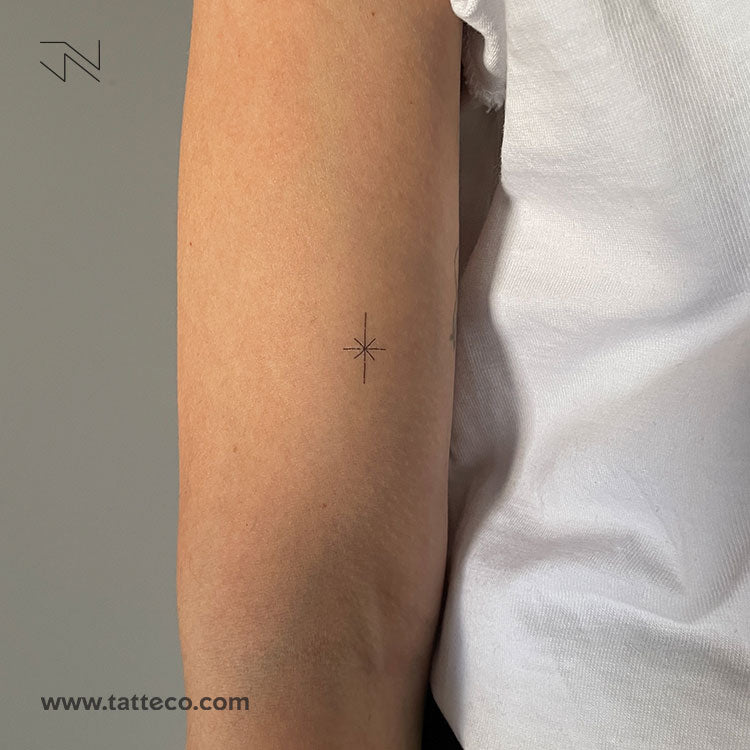The image is an up-close color photograph showing the right upper arm of a person with tan skin, wearing a short-sleeved white cotton t-shirt. Prominently displayed on the arm is a detailed black tattoo consisting of a finely drawn cross with an X at its center, resembling a star shape. Additionally, there are two lines near the upper left corner of the image that look like lightning bolts. The background on the left side is grey. In the bottom left corner, the website URL "www.TATTECO.com" is written in bold black letters. The arm appears to be showcased to demonstrate what the tattoo would look like on the skin.